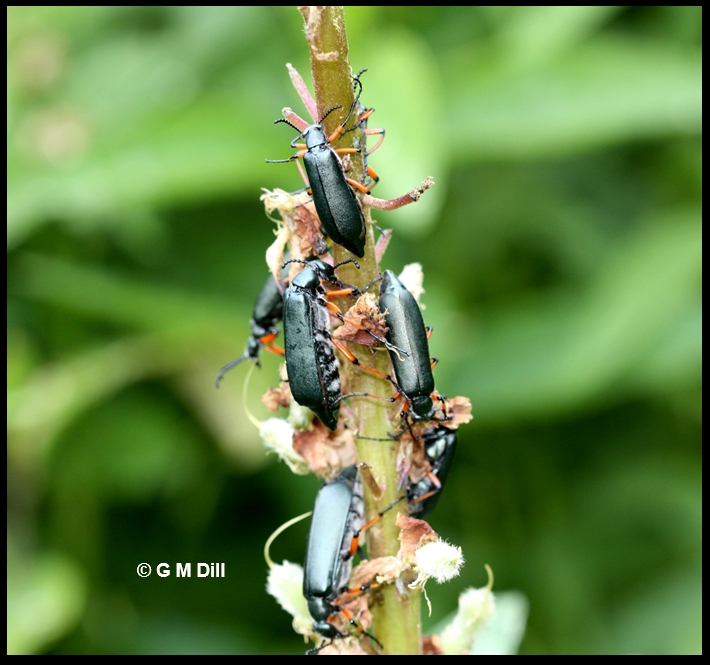In this close-up, daytime photograph, several black insects with orange and black legs and black antennas are captured walking along a green plant stalk. The plant is seen in a horizontal layout, adorned with reddish-pink flowering bits on either side. Of the five beetles, two are facing upwards, while three are positioned with their heads down. The background comprises out-of-focus green leaves, adding to the natural setting. In the bottom left-hand corner of the image, the text reads © GM Dill, marking the photograph with a copyright. The detailed, crisp depiction of the insects and plant contrasts with the blurry foliage in the background, highlighting the intricacies of the foreground subjects.